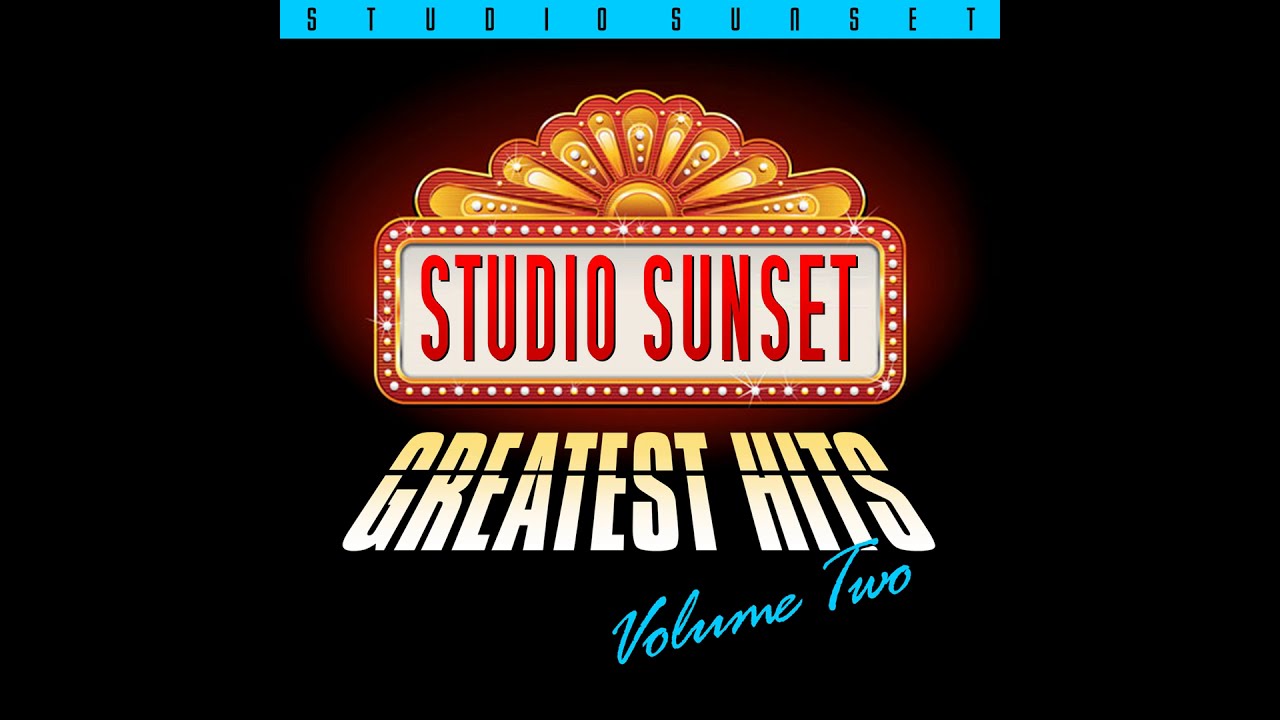This is an image featuring the graphic for "Studio Sunset Greatest Hits Vol. 2." The background is an all-black landscape-oriented canvas. At the very top, there is a blue rectangular banner with the words "Studio Sunset" in black text, closely spaced. Below this, the main focal point resembles a classic theater or Las Vegas marquee sign: "Studio Sunset" is emblazoned in red text on a white backdrop, surrounded by flashing lights that evoke a neon, Broadway-like feel. Above the sign, a sunburst design in shades of orange and red adds a vibrant touch.

Directly below the marquee sign, the words "Greatest Hits" are displayed in a bold, cinematic style reminiscent of the opening crawl in Star Wars, with gradient text fading from white to yellow. Diagonally ascending into the "T" of "Hits," "Volume 2" is elegantly scripted in blue italics. This detailed imagery suggests a promotional piece for a media product—potentially a TV show or a music album—titled "Studio Sunset Greatest Hits Vol. 2."